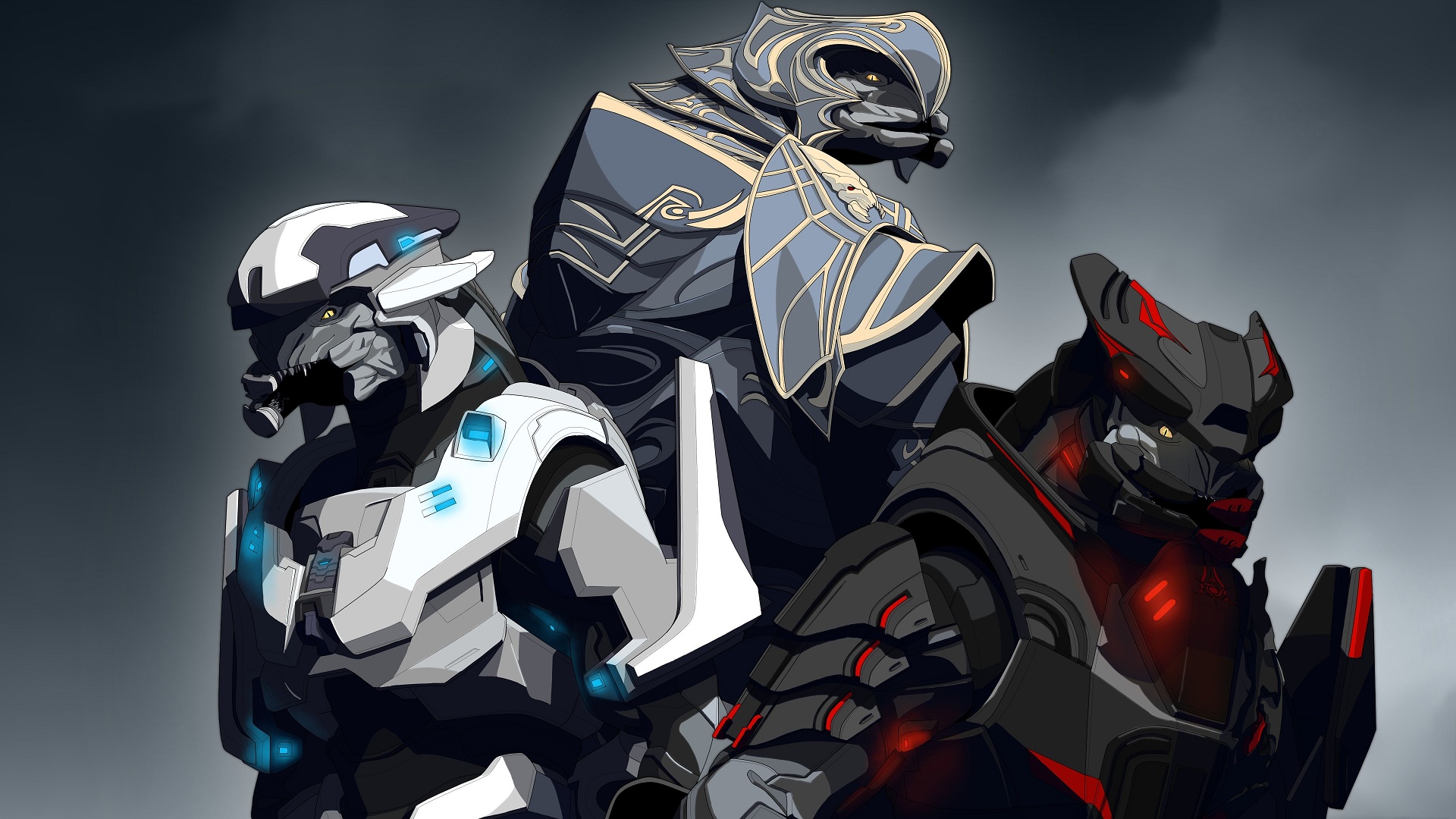In the image, three robotic-looking alien characters are depicted in a 3D cell-shaded style, reminiscent of characters from the Halo video game, posed back-to-back in a triangular formation against a smoky gray background. The central and tallest character, positioned at the top, wears ornate black armor with gold trim, giving a samurai-like appearance, and has a gray alien face with a turtle-like mouth and small yellow eyes. On the left, a shorter character dressed in white armor accented with blue lights and gray trim features a helmet with horn-like protrusions and a green, dinosaur-esque face. The right-most character is clad in menacing gray and black armor with red highlights, exuding an assassin's aura, and also sports a helmet with horn-like details. The background is a dark, smoky gray, adding to the overall mysterious and intense atmosphere.